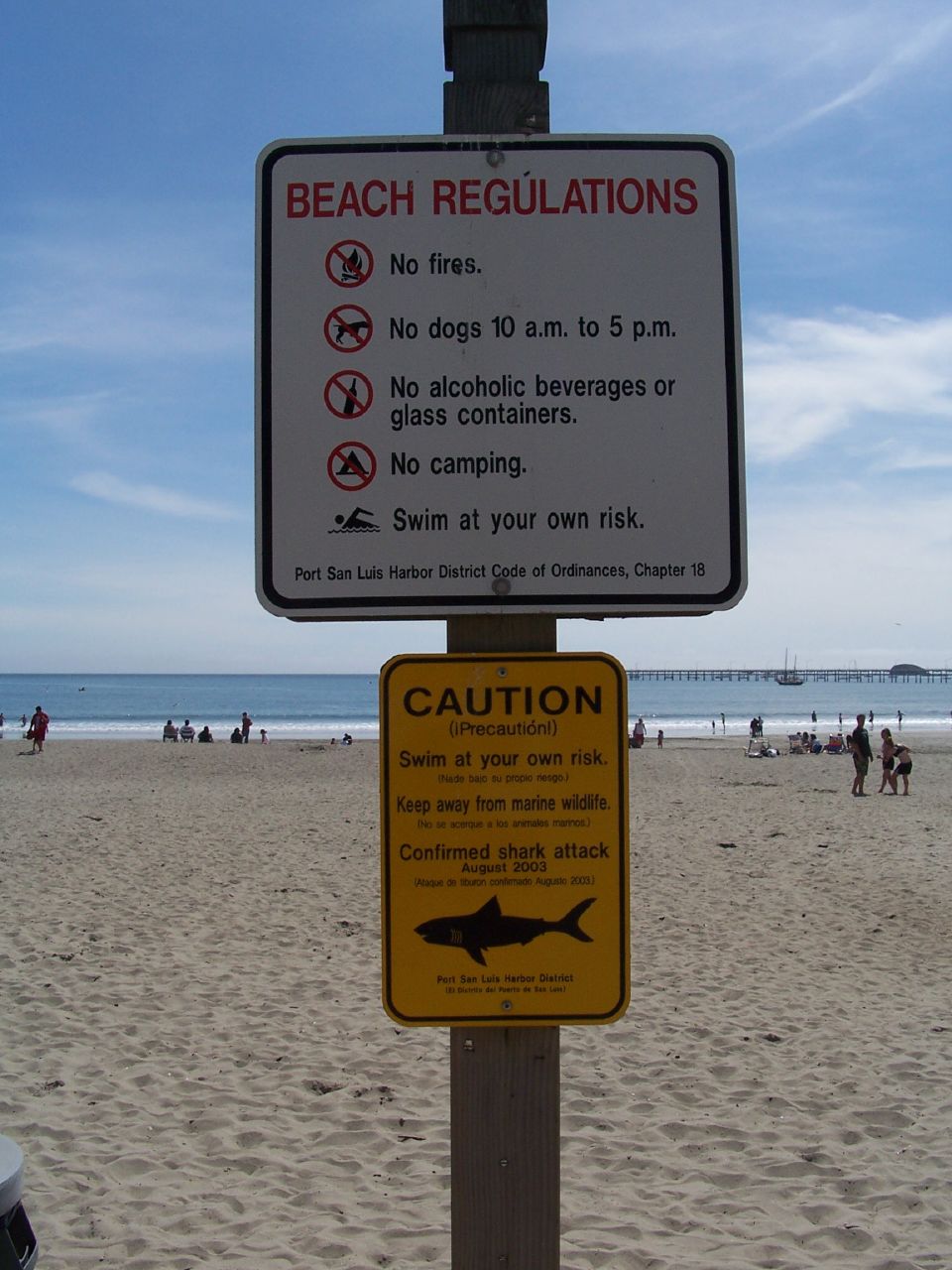In the image, we are positioned in front of a bustling beach with yellow sand, where several people can be seen both onshore and swimming in the ocean's blue waters. The vibrant blue sky above is adorned with wispy white clouds, adding to the scenic beauty. Prominently featured is a wooden signpost to which two signs are affixed.

The top sign is white with a black border, and prominently titled "Beach Regulations" in red text. It features several regulations each accompanied by corresponding icons: a black fire icon with a red circle and diagonal slash indicating "No Fires"; a dog icon with a similar red circle and slash and the text "No Dogs 10 AM to 5 PM"; an alcohol bottle with a red circle and slash, specifying "No Alcoholic Beverages or Glass Containers"; a tent icon with a red circle and slash denoting "No Camping"; and a swimmer icon stating "Swim at Your Own Risk." Additionally, the bottom of the sign references the "Port St. Louis Harbor District Code of Ordinances, Chapter 18."

Below this, the second sign is yellow and serves as a cautionary warning. It bears the text "Swim at Your Own Risk" and "Keep Away from Marine Wildlife," along with a silhouette of a black shark indicating "Confirmed Shark Attack" from August 2003, issued by the "Port St. Louis Harbor District."

The signpost, surrounded by beach activities, serves as a crucial guide ensuring the safety and compliance of beachgoers. In the far background, two boats dot the horizon, completing the picturesque yet informative beach scene.